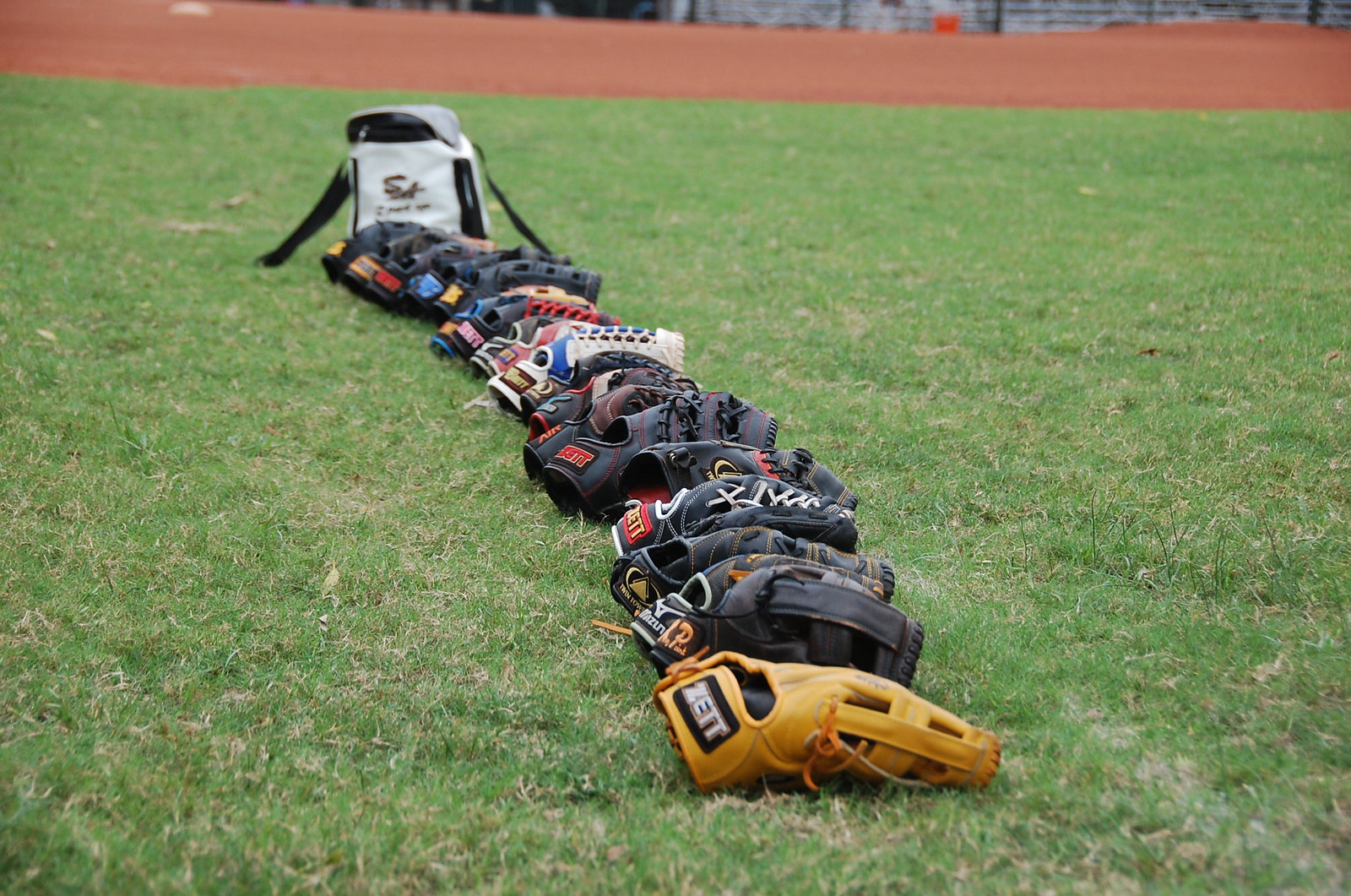The photo features a close-up of various colored baseball mitts meticulously lined up in a single row on a patch of green grass, with some brown dirt spots interspersed. From the front of the line, there's a prominently tan glove followed by several black mitts. In the middle, a white glove stands out before more black mitts eventually lead up to a white bag. The gloves are all positioned with their catching sides down and the tips facing to the right. Each glove, including those in unique colors such as deep yellow, deep blue, light blue, and deep purple, displays a brand name near the cuff area where the hand would enter, including distinguishable brands like Z.E.T.T. The arrangement sits on well-kept grass with visible individual blades and some patches of dried grass, adding texture to the scene. In the background, the brown dirt of a baseball diamond or track subtly contrasts against the vivid green field.